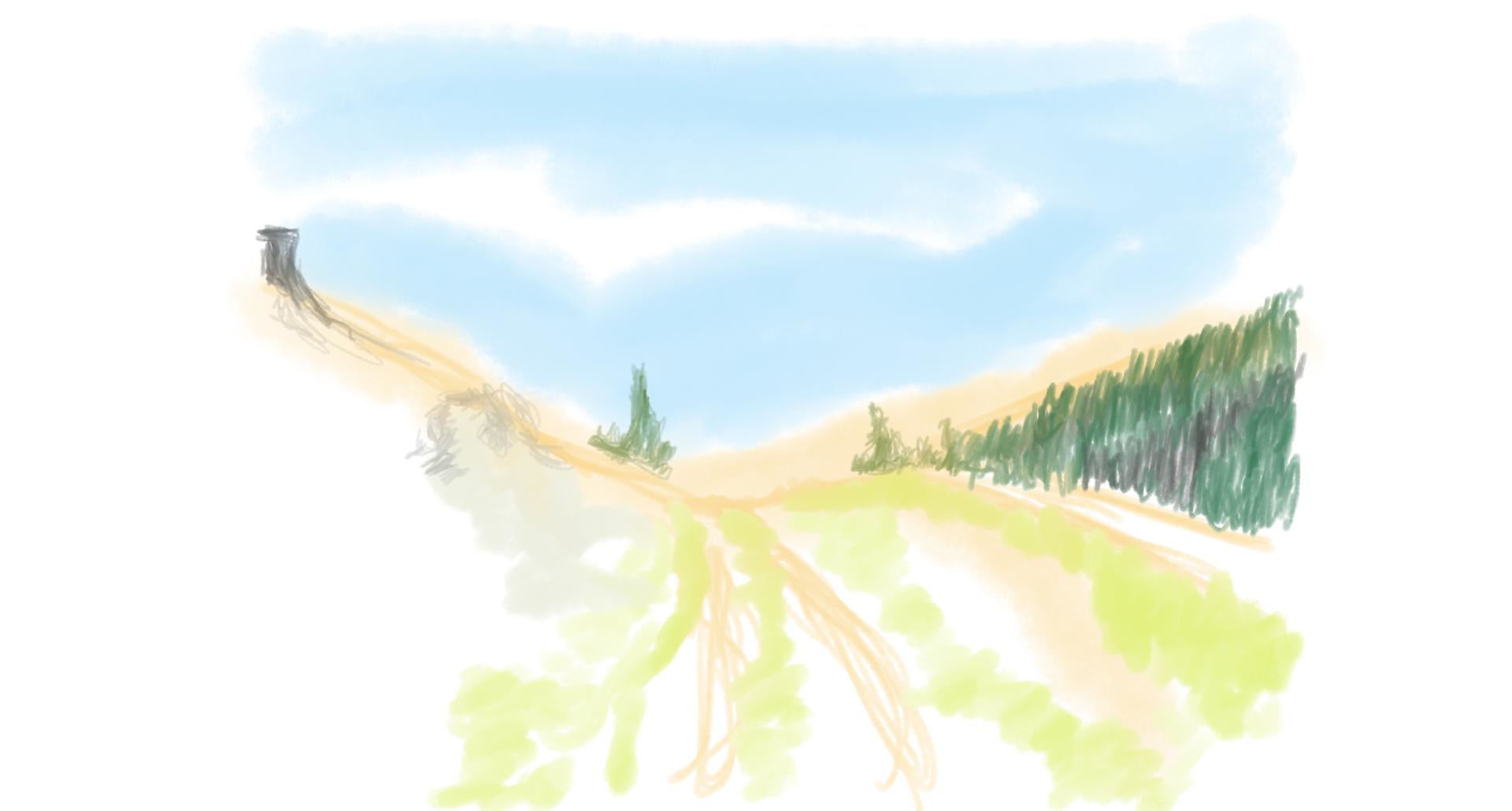This semi-finished artwork appears to be created using pens, crayons, or possibly paint. It depicts a rustic hillside landscape with a roughly sketched road winding up the hill. On the right side of this road, sporadically drawn tall grass forms the primary foliage, while the left side features sparse patches of grass. The sky above is rendered with shades of blue, accented by white areas that effectively convey the presence of clouds floating above the scene. Although the painting lacks polish, it captures the essence of a scenic and rugged hillside journey.